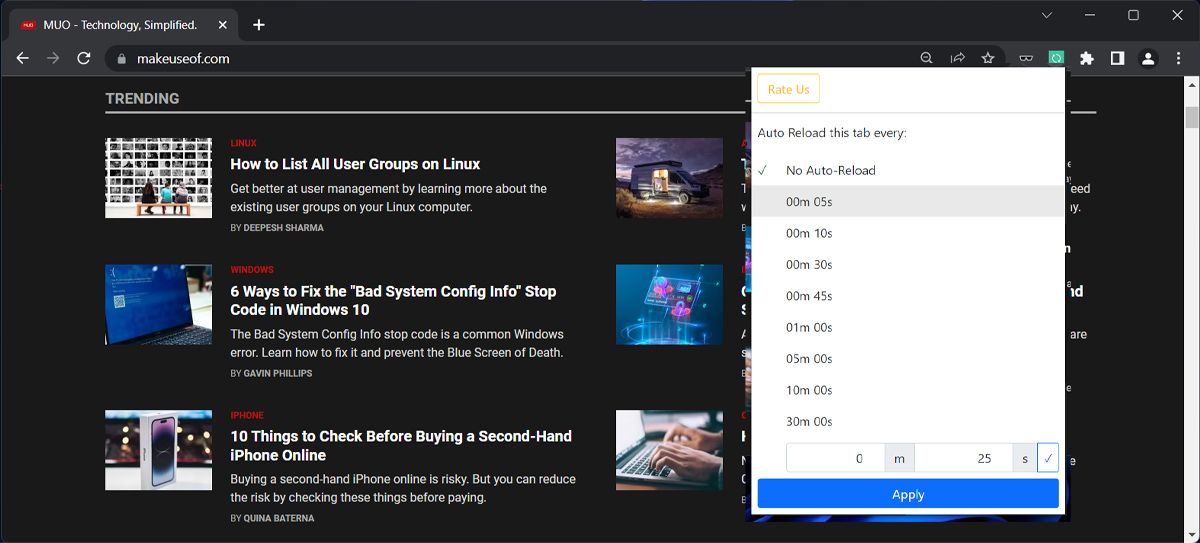The image is a screenshot from the website makeuseof.com, highlighting its "Trending" section. The section features a series of articles accompanied by related images. The first article is titled "How to List All User Groups on Linux," guiding users on improving their management skills by understanding their existing user groups; it is paired with an image of people sitting on a bench. The second article, "Six Ways to Fix the Bad System Config Info Stop Code in Windows 10," aims to assist users in troubleshooting this specific Windows error and includes an image of an open and powered-on laptop. The third article, "Ten Things to Check Before Buying a Second-Hand iPhone Online," offers essential tips to minimize risk when purchasing a used iPhone online, illustrated by an image of an iPhone in its box. Overall, the screenshot encapsulates a variety of tech-related tips and solutions promoted on the website.